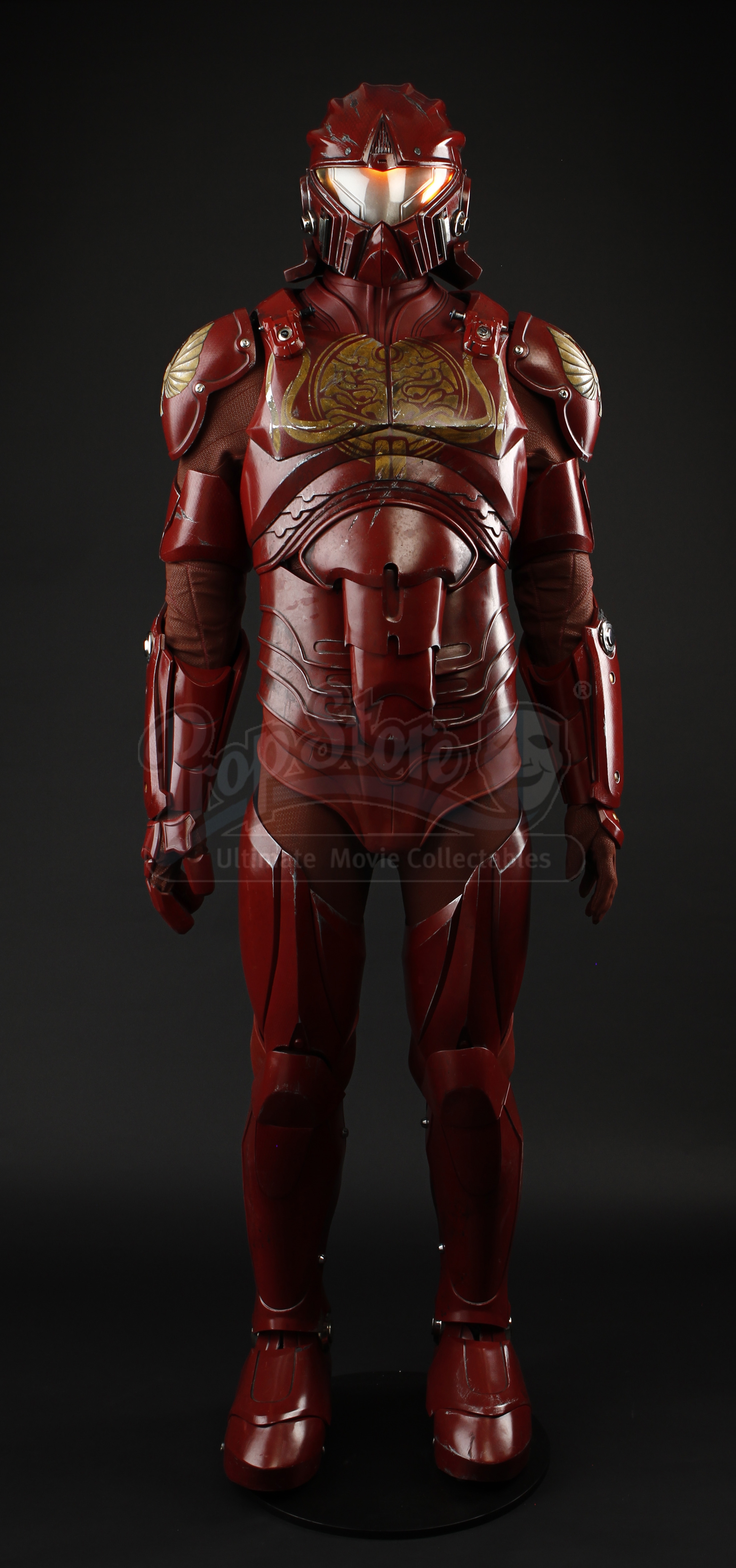The image showcases a narrow, rectangular, color photo of a full-body costume or statue, likely inspired by a fusion of Iron Man and samurai aesthetics. The suit is predominantly a dark burgundy or brick red color, exhibiting a shiny, reflective surface. The helmet has a dark burgundy tone, reminiscent of a samurai helmet, featuring a reflective visor rather than traditional plumes or horns. The costume is thoroughly armored, with segmented, flexible torso armor sections and long gauntlet gloves, ensuring complete coverage of the wearer. The shoulder pads are distinctly styled with Asian design influences, painted gold, and the chest plate also intricately decorated with gold patterns. The legs and boots seamlessly transition from the rest of the suit, maintaining the same shiny, dark burgundy appearance. The costume's detailed design suggests it might be a model or statue fit for display in a museum. Additionally, a white watermark spans across the midsection, partially featuring an unreadable smiling face and some indistinct text.